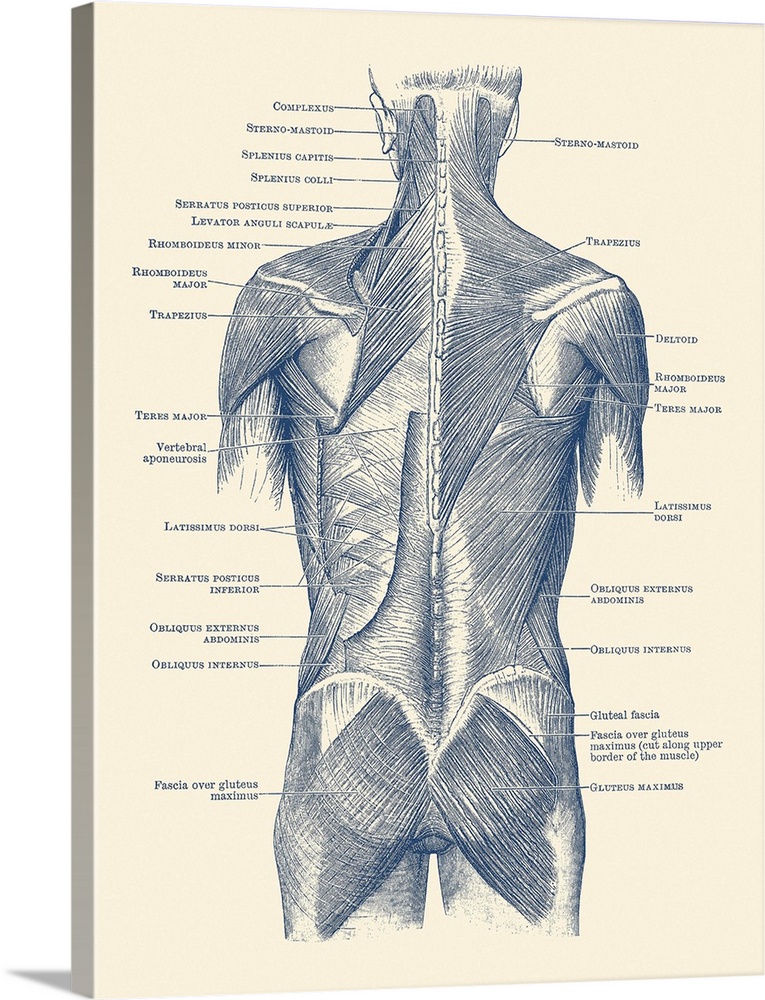This detailed anatomical drawing showcases the muscles of the human back, meticulously rendered with a fine line pen or marker in a dark charcoal gray hue against a beige background. The illustration includes comprehensive labeling of each muscle, extending from the lower part of the head and ears, down the neck and shoulders, across the upper and middle back, and continuing to the buttocks and top of the legs. Prominent muscles such as the trapezius, triceps, shoulder blades, and gluteus maximus are clearly visible, along with the spinal area, highlighting multiple layers of muscular structure.